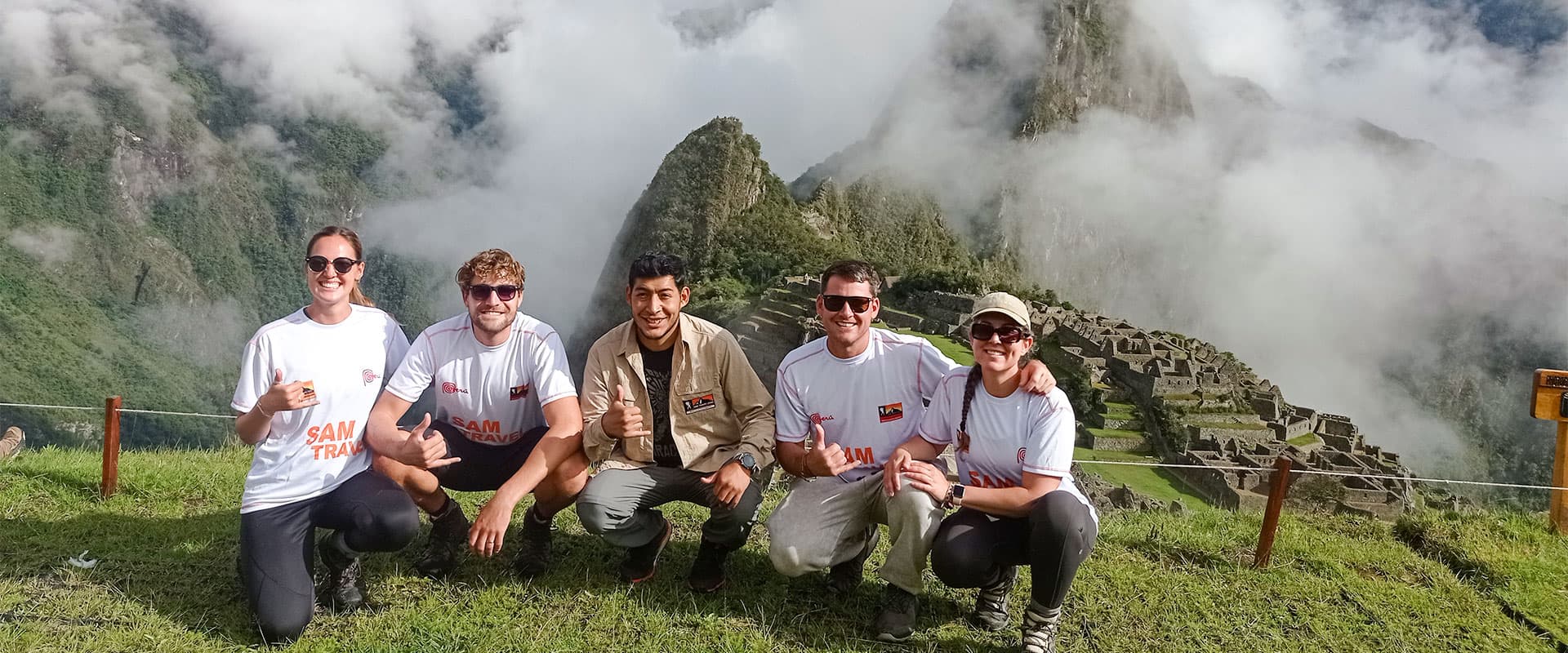This vibrant image captures a group of five individuals posing amidst the lush greenery of a hilltop or mountaintop, with a stunning backdrop of Machu Picchu's ancient stone ruins. Kneeling on the grassy terrain, they exude a sense of adventure and camaraderie. Behind them, slender wooden stakes connected by a thin string mark the edge of a drop-off, adding a hint of thrill to the scene. Swirling clouds and dense fog envelop the majestic mountains in the background, creating the illusion that they are high up in the clouds. 

In their white "Sam Travel" T-shirts, the group consists of two women and three men, all donning sunglasses except for the man at the center who stands out in a tan jacket over his shirt. Noteworthy are the stone monuments and stairs to their right, hinting at the historical richness of their location. They all display cheerful expressions, some making gestures with their hands, except for the woman on the far right. On this sunny day, their playful shadows stretch to the left, adding depth to the photo. A partially visible yellow sign peaks in on the far right of the image. The closeness of the young man and woman on the right suggests they might be a couple, with his arm gently wrapped around her, enhancing the heartwarming feel of this tourist snapshot.